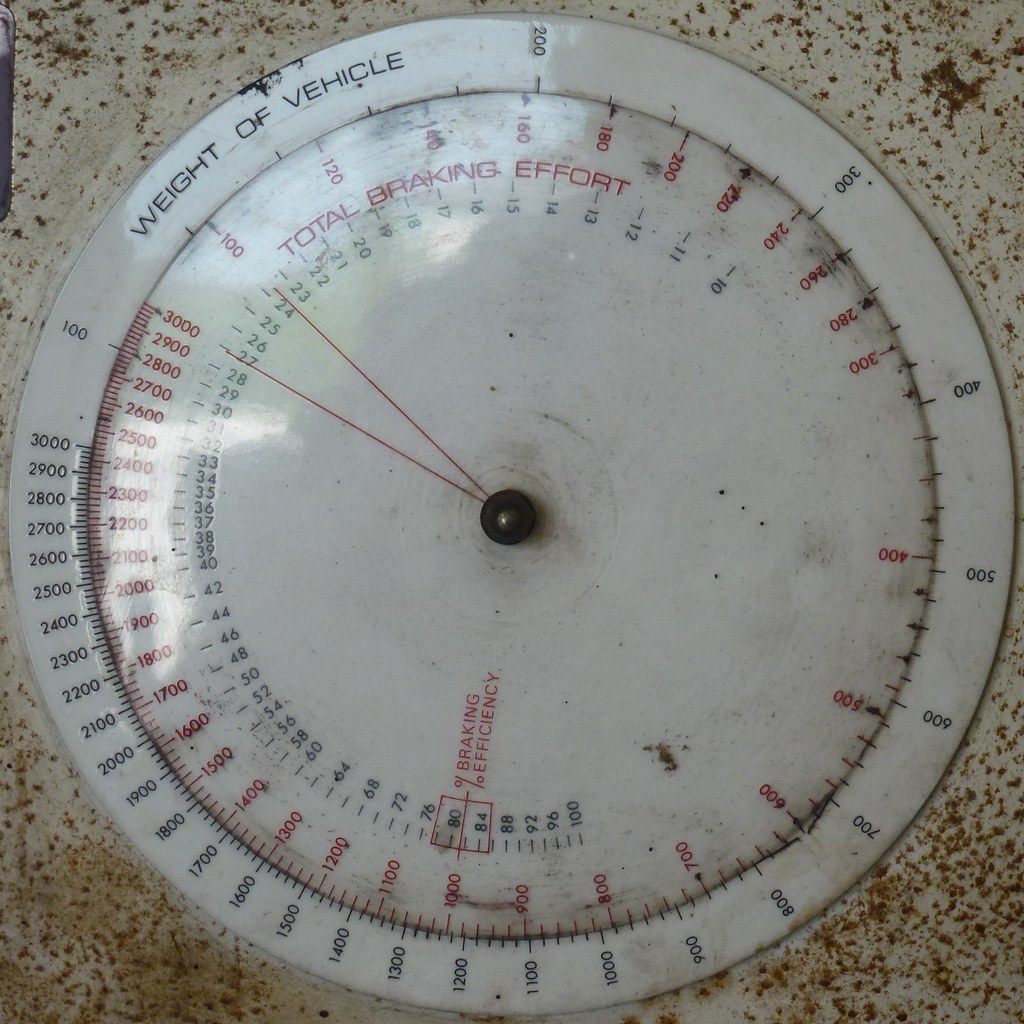The image features an old, white dial embedded in a slightly rusty metal surface. The outer rim of the dial bears the words "weight of vehicle" and showcases black numbers ranging from 100 to 3,000 in a clockwise direction, becoming closer together as they approach 3,000. The white face of the dial includes a beveled border with additional red text in the center displaying "total braking effort" and "percentage of braking efficiency." Two inner dials provide specific readings, with one indicating total braking effort and another bracketed area at the bottom denoting the percentage of braking efficiency. This scale appears aged, with visible rust and discoloration at the corners, giving it a worn and dirty appearance.